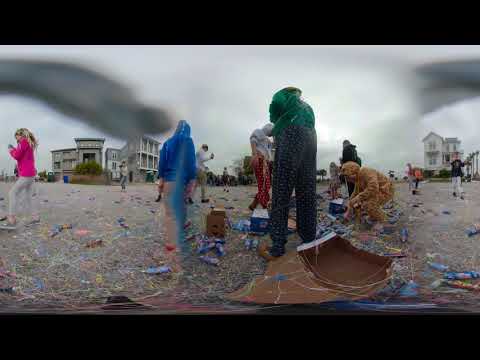This full-color, horizontally rectangular photograph, with a black band across the top and bottom, captures a somewhat blurred outdoor scene on an overcast day with a gray, cloudy sky. The image appears to be taken on a beach, evidenced by the possibly pebbled or sandy ground. Several young people, dressed in full pants and hooded jackets, possibly resembling hazmat suits or costumes, are scattered throughout the open area. They are diligently bent over, picking up various debris, post-cleanup of what seems like a festive event, possibly involving a piñata or fireworks. Strewn across the ground are colorful materials that look like silly string, confetti, and streamers in vibrant hues of yellow, blue, orange, and more. Cardboard boxes and blue bottles, which could be water or beer bottles, are also visible. In the background, a few large, multi-story houses with columns stand, adding a sense of depth to the image. The overall scene conveys the sense of a concerted cleanup effort in a chilly, post-celebration environment.